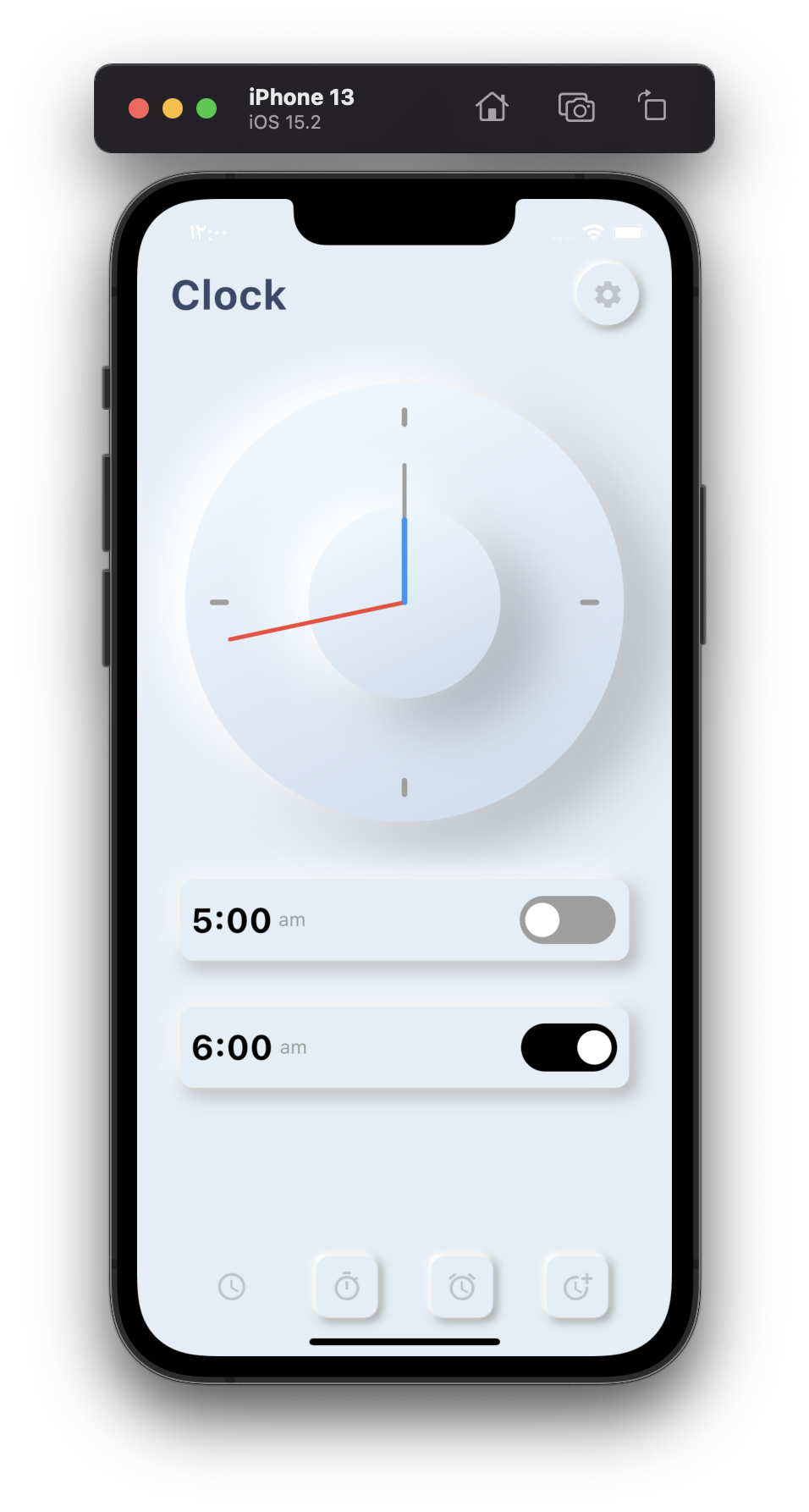This image features a sleek black iPhone 13 prominently displayed against a plain background. The device is centered on the page with its buttons clearly visible on both the left and right sides.

Directly above the iPhone is a standalone panel, appearing like a cropped image of the phone's home screen, which should normally be at the bottom of the phone. This panel showcases the iPhone's Clock app set against a gray background. At the top left corner of this screen, "Clock" is written in bold black letters, while a gray cogwheel icon is positioned to the right of the title.

In the center of the screen is a large, round clock face with a raised middle. The clock's hour hand points to 12, and the minute hand is nearly at the 45-minute mark. A glowing effect highlights the area from 45 to 12, contrasting with a shaded effect that covers the rest of the clock face.

Below the clock face, two alarm settings are displayed. The first alarm is set for 5 a.m., and its toggle switch on the right is in the off position. Directly beneath this, another alarm is set for 6 a.m., with its toggle switch turned on.

At the bottom of the screen, there are four distinct buttons. The leftmost button is labeled "Clock" and lies flat against the page. The next three buttons, which are raised, from left to right include the Timer, Alarm, and a refresh-looking icon.

This detailed depiction provides a thorough visual description of the iPhone 13 and its Clock app interface.